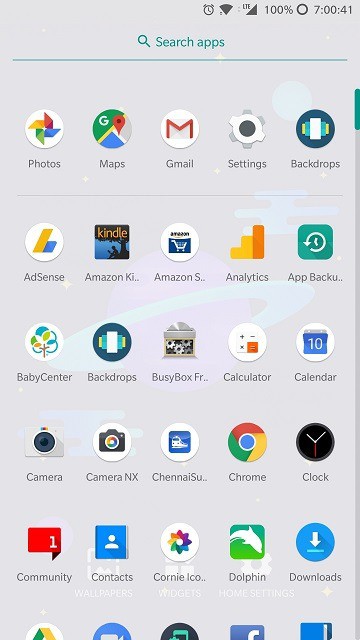A detailed caption for the image:

The image displays a smartphone screen showcasing a neatly arranged grid of applications. The screen's background is gray, featuring a subtle, planetary-themed design with faint outlines of planets and various shapes scattered across the backdrop. At the top of the screen, the status bar indicates a fully charged battery at 100%, and the time is precisely 7:00:41. Immediately beneath the status bar, a teal-colored text field reads "Search apps," accentuated by a teal underline.

The main portion of the image is occupied by six visible rows of app icons, the bottom row slightly cut off by the screen's edge. Most app icons are circular, with a few square ones interspersed. The top row includes icons for Photos, Maps, Gmail, Settings, and Backdrops. The second row contains AdSense, Amazon Kindle, Amazon Shopping, Analytics, and App Backview. The third row features Baby Center, Backdrops once again, BusyBox, FR, Calculator, and Calendar. Each app icon is clearly displayed, making it easy to discern the array of tools and utilities available to the phone's user.